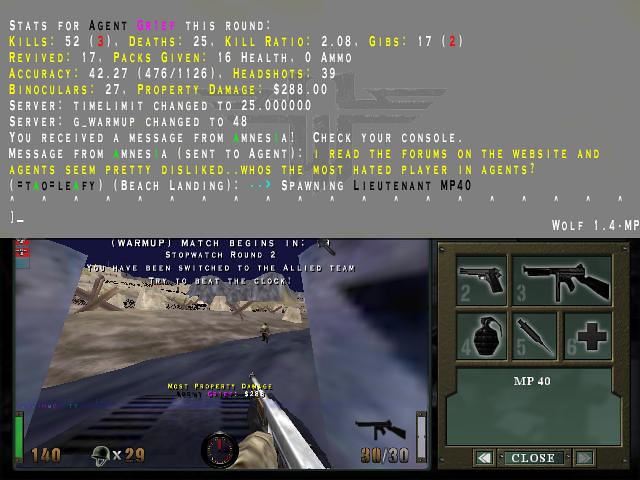The image is a horizontally rectangular screenshot from a video game. The upper half of the frame features a gray background displaying several lines of game-related information in a variety of colors including white, yellow, black, with occasional spots of pink and red. The lower half contains the actual gameplay area, which is also predominantly gray. Emerging from the bottom of the gameplay area is a hand holding a gun, with the barrel aimed towards the center of the frame. To the right side of the lower half, there's a rectangular box showcasing various weapons.